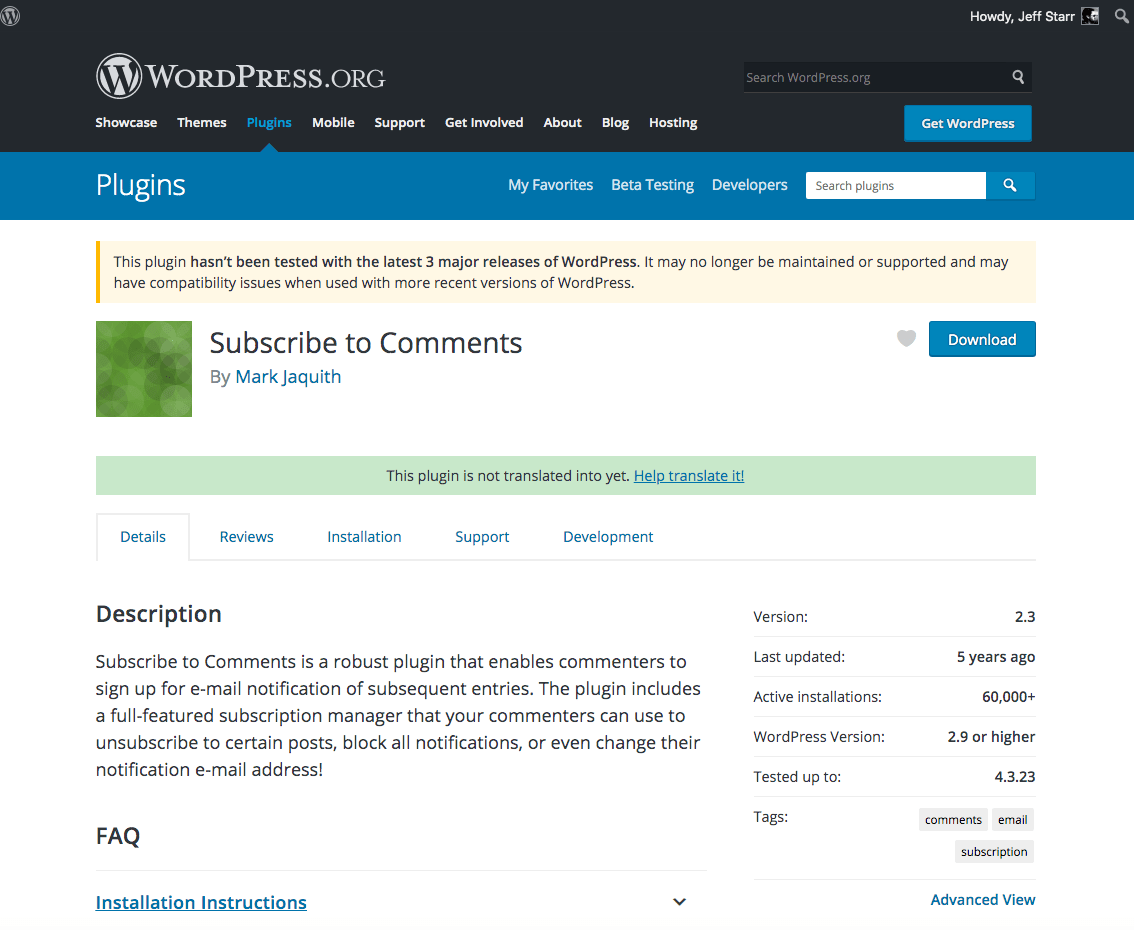The image depicts the WordPress.org website interface. At the top, there is a prominent logo consisting of a large "W" inside a white circle. Below the logo, there is a navigation menu with the options: Showcase, Themes, Plugins, Mobile, Support, Get Involved, About, Blog, and Hosting. On the right-hand side, there is a blue bar with the prompt "Get WordPress."

In the header section, there's a search bar labeled "Search WordPress.org." Adjacent to this, a user greeting appears, saying "Howdy, Jeff Star." Below the greeting, a notification reads "Subscribe to Comments by Mark Jaquith."

Towards the right side, there is a blue download button accompanied by a warning message stating, “This plugin hasn't been tested with the latest three major releases of WordPress. It may no longer be maintained or supported and may have compatibility issues when used with more recent versions of WordPress.”

Further down, there is a section indicating that "This plugin is not translated into yet. Help translate it," with an interactive option to click for translation.

The page also includes a detailed description of the plugin, "Subscribe to Comments," which is described as a robust plugin that allows commenters to sign up for email notifications of subsequent entries. It mentions the ability to block notifications or change the notification email address.

In addition, the page features FAQ sections beginning with "Installation Instructions," which is an expandable item for more details.

On the right side of the page, there are specifications listed, including Version, Last Updated, Active Installations, Tested up to, and Tags.